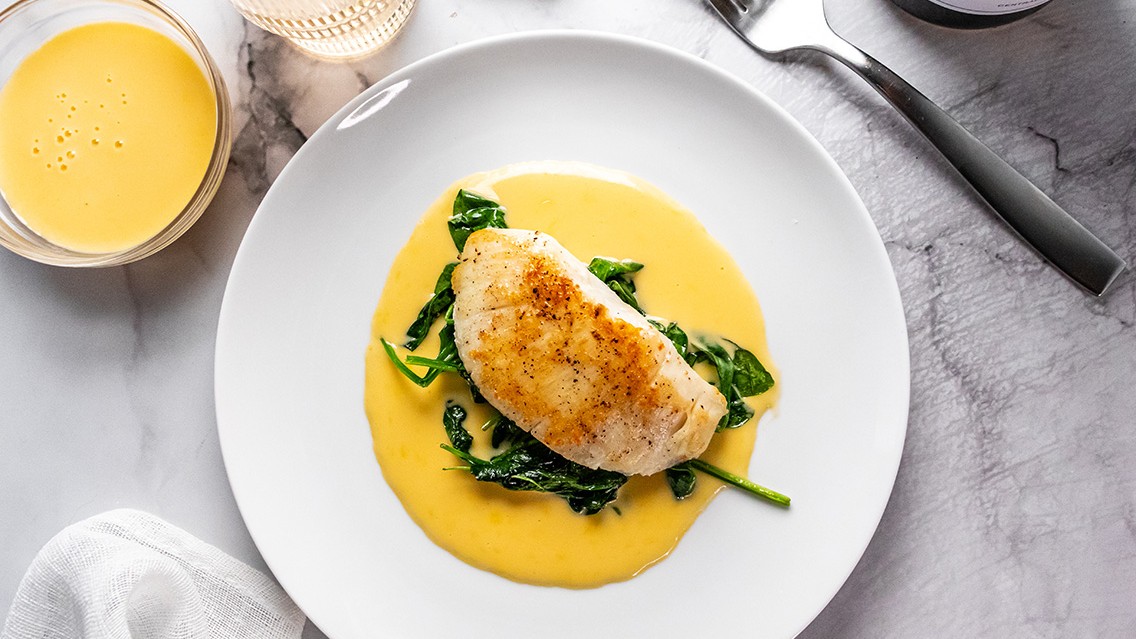The image showcases a beautifully plated dish on a white porcelain plate, placed on a marble countertop. The main focus is a piece of grilled chicken breast, browned and seared to perfection, resting atop a bed of wilted spinach, all drenched in a rich, yellow hollandaise sauce. To the right of the plate, a silver fork is neatly positioned, and a white fabric napkin is elegantly placed to the left. In the upper left corner of the image, a small clear bowl holds additional hollandaise sauce, exhibiting slight bubbling. Just beside it, a glass of water sits partially visible. The composition of the scene is brightly illuminated, highlighting the textures and rich colors of the dish and its accompaniments.